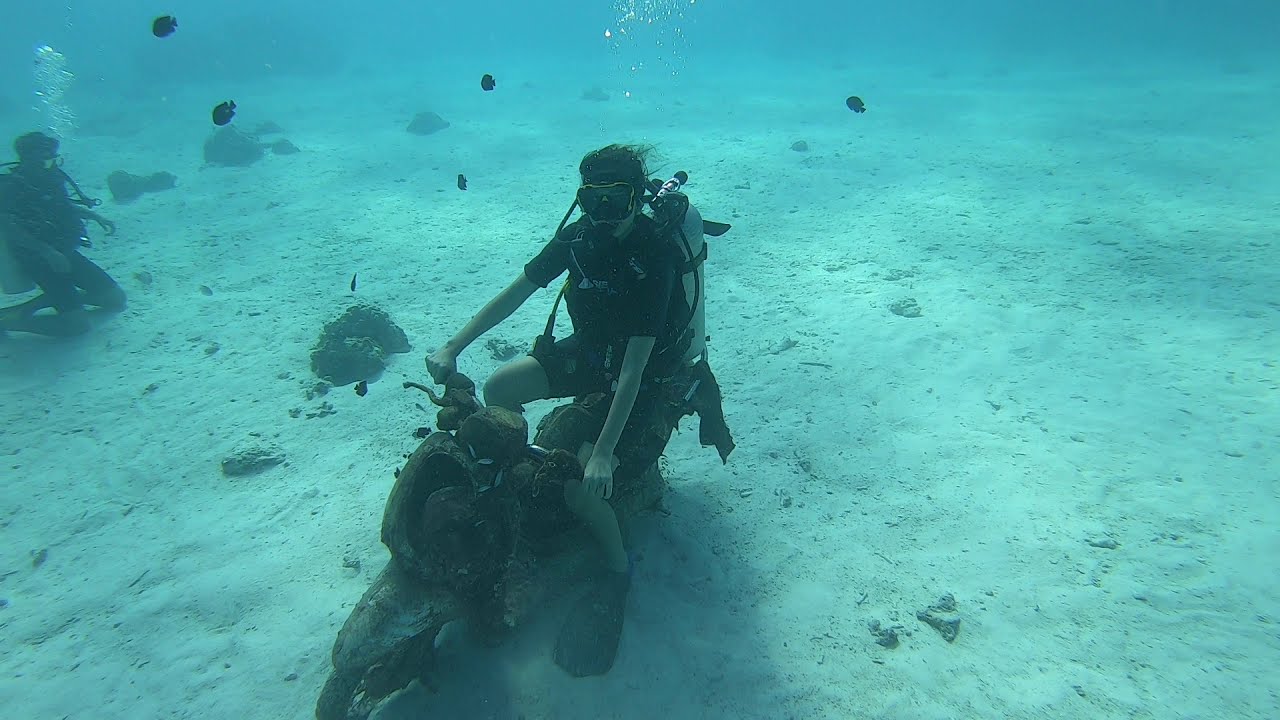Underwater, in a pale aqua expanse possibly within an ocean or lake, a detailed tableau unfolds. A man in full scuba gear, including black shorts, a black short-sleeved top, goggles, and an oxygen tank, sits atop a very old, rusted motorcycle that has almost fossilized over time, showing signs of age and perhaps stone encrustation. Attached to the motorcycle or to the diver himself, a flag waves gently in the water. To the left of this scene, another scuba diver kneels on the sandy ocean floor, surrounded by scattered rocks and exhaling a stream of bubbles. Fish swim leisurely between the two men, adding life and movement to the underwater stillness. Rocks and sand cover the sea bed, contributing to the overall sense of time standing still in this submerged world.